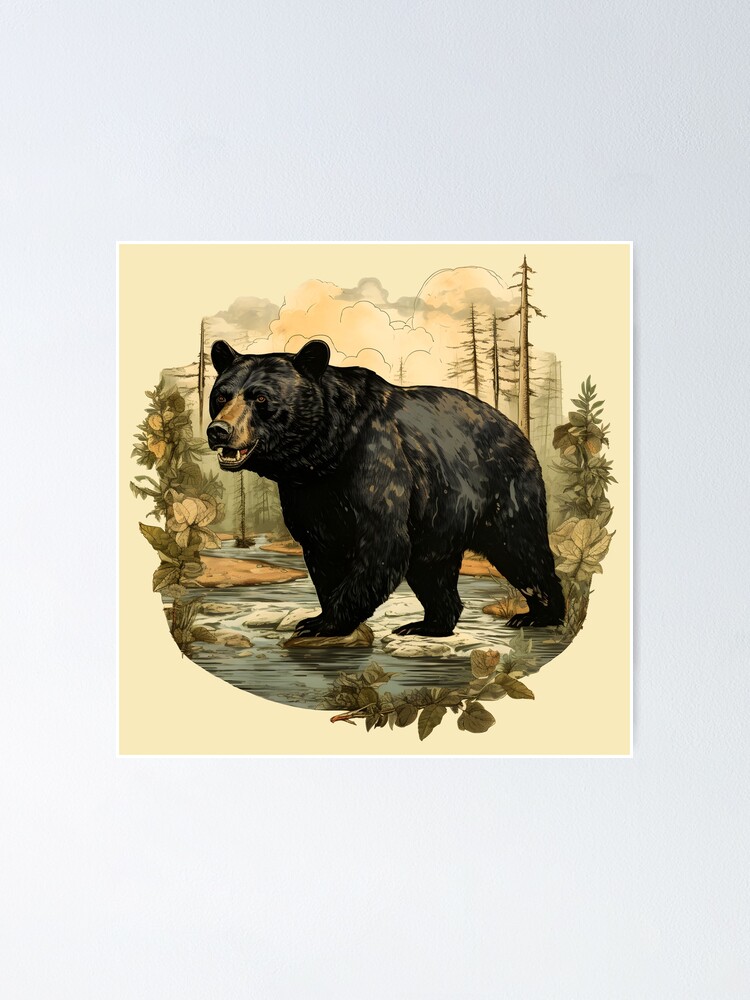This oil-style painting prominently features a black bear with subtle brown undertones. The bear's snout is a tawny color, and its mouth is partially open, revealing a black nose and some teeth. The bear is depicted walking across light-colored stones in a body of water that has a bluish-gray hue. Surrounding the scene are green leaves and various trees, some looking barren, while others are more lush. In the background, abstract clouds in shades of tan, orange, and gray fill the sky. More trees and a dirt riverbank are also visible in the distance. The entire scene is encapsulated within a circular shape, set against an off-white canvas, adding a unique framing to the composition.